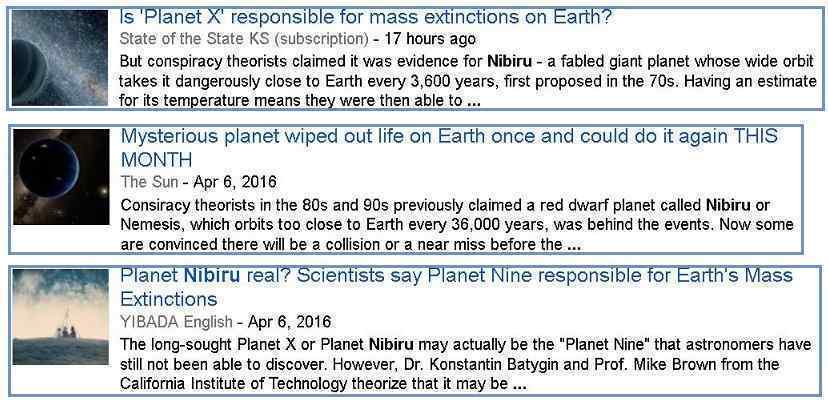This image is a compilation of screenshots from three articles discussing the controversial topic of a mysterious celestial body known as Planet X or Nibiru. The first article, titled "Is Planet X Responsible for Mass Extinctions on Earth?" by State of the State, KS Subscription, published 17 hours ago, explores the conspiracy theory that posits the existence of Nibiru, a gigantic planet with an orbit that brings it perilously close to Earth every 3,600 years. This theory emerged in the 1970s, suggesting that understanding its temperature is crucial for further study.

The second article, from The Sun dated April 6, 2016, is headlined "Mysterious Planet Wiped Out Life on Earth Once and Could Do It Again This Month." It recounts claims from conspiracists in the 1980s and 1990s who believed that a red dwarf planet named Nibiru or Nemesis, which approaches Earth every 36,000 years, was responsible for catastrophic events. Some theorists now fear an imminent collision or near-miss.

The third article, titled "Planet Nibiru Real? Scientists Say Planet Nine Responsible for Earth's Mass Extinctions," from Ibada English on April 6, 2016, considers the possibility that the elusive Planet X or Nibiru could actually be Planet Nine, an hypothesized planet that astronomers, including Dr. Konstantin Batygin and Professor Mike Brown from the California Institute of Technology, have yet to discover.